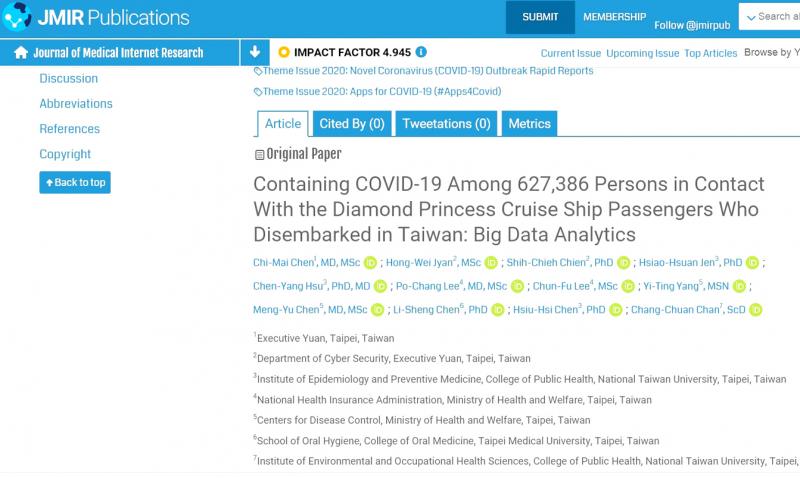The image features a website layout with a light blue header. Positioned centrally in the top section is a globe in a lighter blue hue, adorned with abstract black continents. Prominently displayed above the globe is bold, all-caps white text that reads "JMIR," followed by the word "Publications." 

On the right side of the header, there's a darker blue button with white text labeled "Submit." Following this button are sections labeled "Membership" and "Follow @JMIRPub." Positioned in the upper-right corner is a white search button accented with blue text.

Below the blue header, on the left side, the background transitions to a solid blue with white text. Here, there's an icon of a house next to the name "Journal of Medical Internet Research." Further down on a white background, blue text provides links to "Discuss," "Abbreviations," "References," and "Copyright."

A blue button with white text labeled "Back to Top" is located towards the bottom of the layout. On the right side, a grey section highlights COVID-related content, including an area labeled "Articles Cited by Tweeted Notions" followed by "Metrics."

The main body of the page is white with black text and features an "Original Paper" titled "Containing COVID-19 Among 627,386 Persons in Contact with Diamond Princess Cruise Ship Passengers Who Have Disembarked from Taiwan: Big Analysis." The section includes a list of contributing doctors and numerous citations from Taiwan.